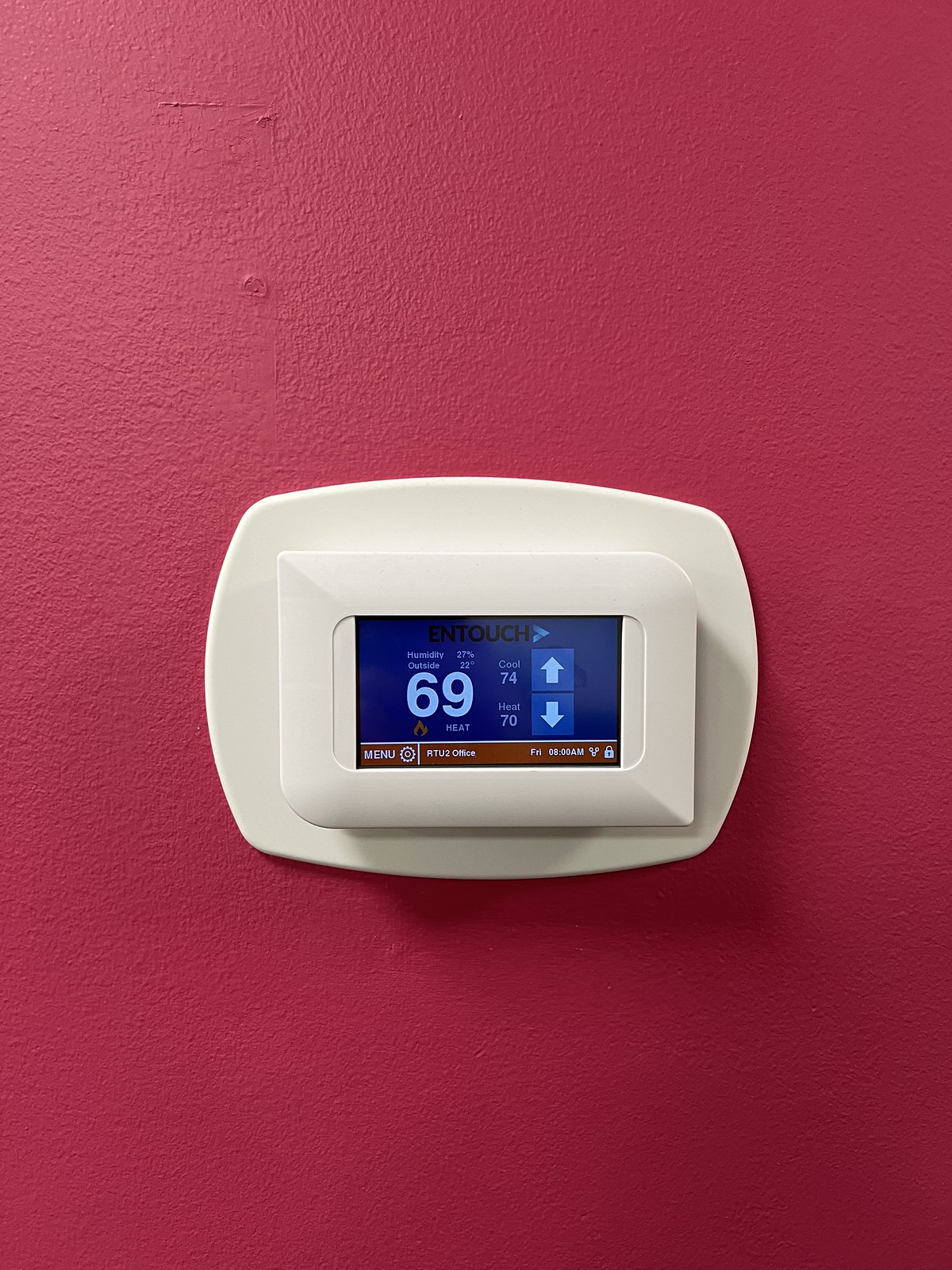In the image, a digital thermostat is prominently displayed, resembling those commonly found in homes or office buildings. The thermostat is mounted on a rounded rectangular plastic plate, both of which are cream-colored. The thermostat itself is a more pronounced rectangular shape, blending seamlessly with its mounting plate.

The screen of the thermostat showcases the brand name "InTouch" (spelled out as E-N-T-O-U-C-H). It features arrow buttons for increasing or decreasing settings. The current temperature is displayed as 69°F, and the system is set to 'heat.' Additional information on the display indicates that the cooling temperature is set to 74°F and the heating temperature to 70°F. At the bottom of the display, a red bar contains the word "menu" accompanied by a settings icon. There is also unreadable text towards the far right corner, alongside a lock icon.

The thermostat is affixed to a vibrant reddish-pink wall, which appears to be painted over drywall. The wall has visible imperfections, with small white nicks and scuffs marring the painted surface, adding a touch of lived-in character to the setting.